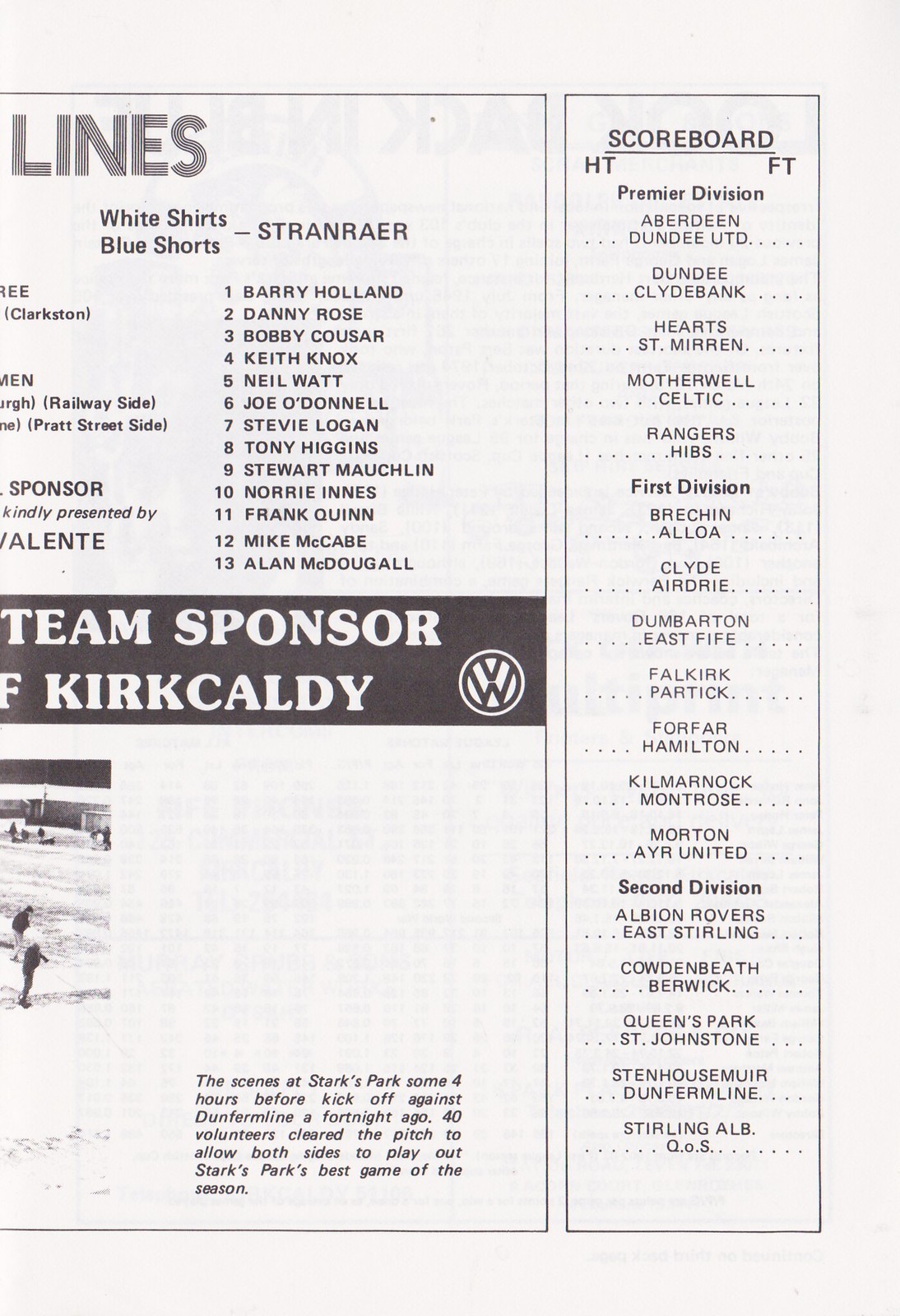The image is a partially cut-off informational sheet for a soccer team, featuring various details about matches and players. The sheet has a grayish background. On the left side, which appears to be cut off, you can see the names of 13 team players: Barry Holland, Danny Rose, Bobby Kuzar, Keith Knox, Neal Watt, Joe O'Donnell, Steve Logan, Tony Higgins, Stuart Bonkling, Murray Inez, Frank Quinn, Mike McAvey, and Alan McDougal. Next to the names, there's a note about their uniform—White Shirts and Blue Shorts—and the team's sponsor, Kirkcaldy Volkswagen.

The center section of the sheet mentions a "Team Sponsor: F. Kirk Gauldy" and features a caption beneath a partial image that reads, "The scenes at Starks Park some four hours before kickoff against Dunfermline a fortnight ago. Forty volunteers cleared the pitch to allow both sides to play out Starks Park's best game of the season."

On the right side of the sheet, there is a vertical box containing a scoreboard with columns labeled HT and FT. The scoreboard lists various soccer matches categorized by division. The Premier Division includes teams such as Aberdeen, Dundee UTD, Dundee, Clydebank, Hearts, St. Miren, Motherwell, Celtic, Rangers, and Hibs. The First Division features Brechin, Alloa, Clyde, Airdrie, Dumbarton, East Fife, Falkirk, Partick, Forfar, Hamilton, Kilmarnock, Montrose, Morton, and Ayr United. The Second Division lists Albion Rovers, East Stirling, Cowdenbeath, Berwick, Queens Park, St. Johnstone, Stenhousemuir, Dunfermline, Stirling Albion, and QOS.